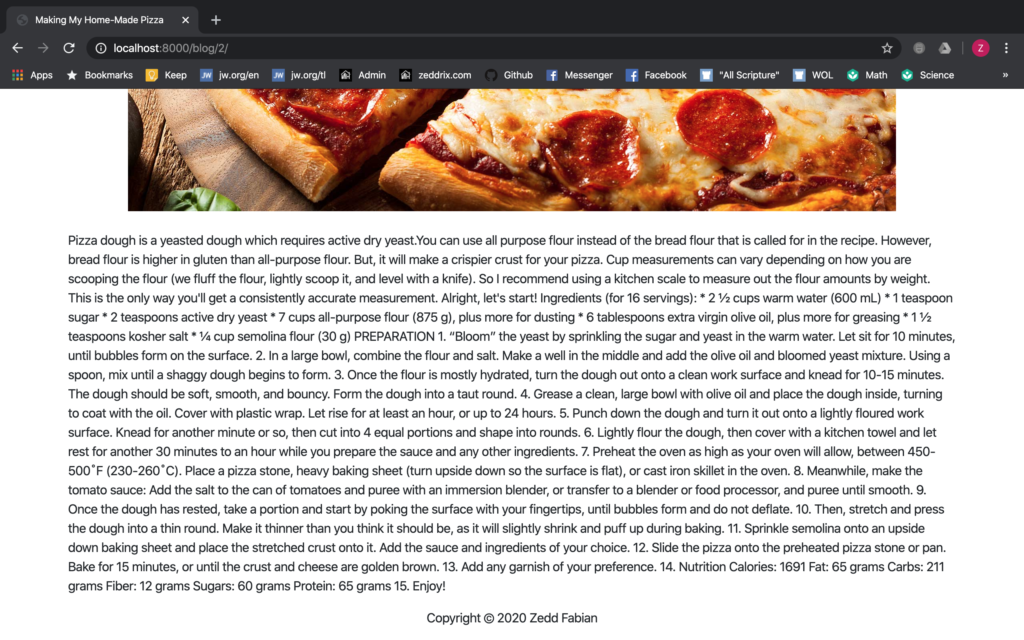A screenshot of a web page is displayed, presenting a detailed blog entry titled "Making My Homemade Pizza." The web page is framed by a sleek black banner at the top, which features a white globe icon and the title text. Navigation buttons, including back, forward, and reload, are visible. The URL indicates the blog is hosted locally at "localhost:8000/blog/2," and there is a star icon for favoriting the page.

In the upper right corner, a profile icon represented by a red circle with the letter "Z" is displayed. The web browser's tabs include "Apps" shown in a colorful dotted pattern, "Bookmarks" denoted by a star, and "Keep." Various bookmarked links are noticed, such as JW.org (listed twice), "Admin," "Zedrix.com," "GitHub," "Facebook Messenger," "Facebook," "All Scripture," "WOL," "Math," and "Science."

The main body of the page contains a partially visible photograph, which seems to be cut off or scrolled down halfway. The photo captures a pepperoni pizza set on a circular wooden board, complemented by a single basil leaf in the bottom portion of the image. The article text below provides a detailed explanation of how to make homemade pizza, although specific details are not visible in this snippet.